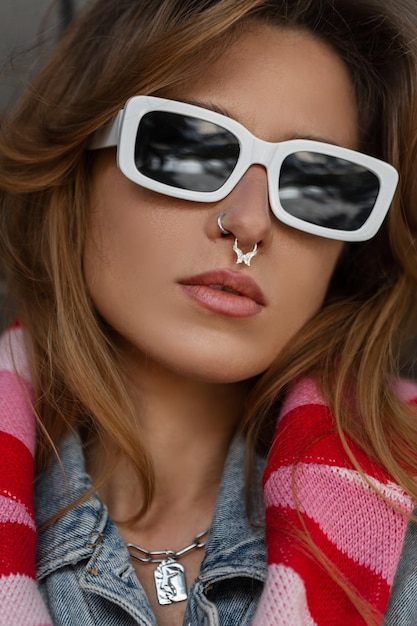This close-up portrait photograph captures an attractive young woman with flawless, smooth skin and defined, plump lips enhanced by pink lipstick and neatly outlined with lip liner. She has light brown, almost auburn, wavy hair that cascades from her head. Her stylish look is accentuated by two nose piercings: a silver ring through her right nostril and a golden septum ring. Donning large, white-rimmed sunglasses with dark lenses that reflect a hint of light, her eyes remain concealed, with only a sliver of her well-groomed eyebrows visible above the frames.

Around her neck, she wears a vibrant pink, red, and white scarf artfully draped over a denim jacket, the latter partially visible due to the close framing of the head-and-shoulders shot. A silver necklace with a pendant lies elegantly against her skin, adding a subtly sophisticated touch to her ensemble. Overall, the image portrays a meticulously groomed, fashion-conscious woman exuding a chic, yet casual vibe.